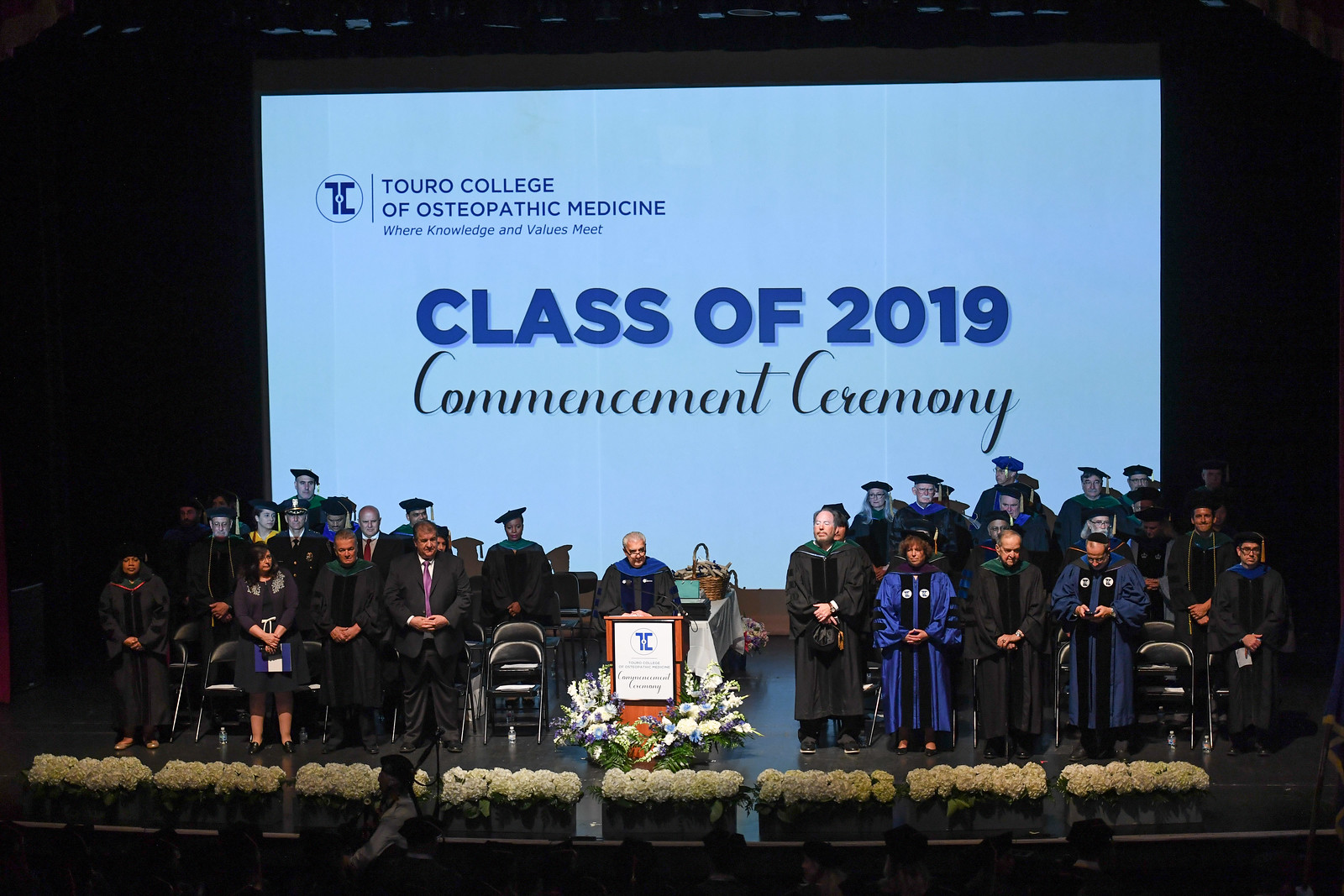The photograph captures a vibrant graduation ceremony for the Toro College of Osteopathic Medicine, held on a stage lined with white flower arrangements. The centerpiece of the stage is a dignified brown wooden podium, adorned with a white and blue sign and surrounded by beautiful bouquets of flowers. A man, clad in a black robe with a blue collar, stands at the podium delivering a speech into a fixed microphone. Graduates, donning black and white robes with traditional caps, are both seated and standing on stage, alongside some dignitaries who are dressed in formal attire. The backdrop of the stage features a large screen projecting the college's logo, accompanied by the motto "Where Knowledge and Values Meet." The display prominently reads, "Class of 2019 Commencement Ceremony" in bold fonts. Additionally, the stage area is illuminated by ceiling lights, contributing to the formal yet celebratory atmosphere. Below the stage, a cameraman captures the moment while other attendees observe attentively.